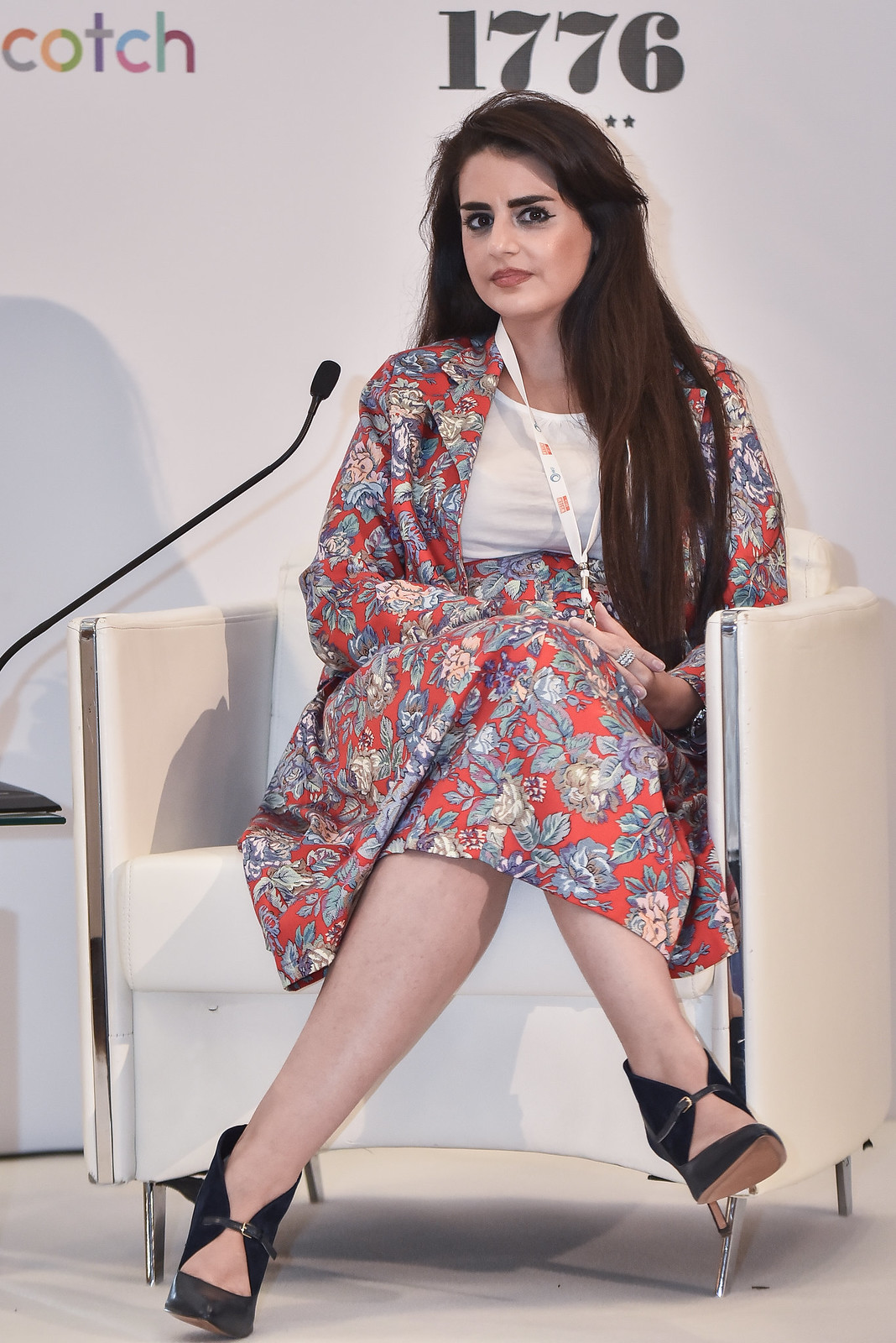The image features a woman of South Asian descent with long, flowing, dark hair that cascades down to her waist, transitioning from black at the top to brown. She is seated on a sleek, modern white chair with silver legs and thick cushions. The woman exudes sophistication as she poses with her left forearm resting on her right leg and her hands gently clasped. Her face, turned at a slight angle, reveals her light brown complexion and expressive, doe-like eyes enhanced with prominent makeup. She is attired in a fashionable red outfit adorned with gray and white floral patterns, consisting of a flattering dress and top, paired with a white blouse underneath. A white identification tag hangs around her neck, complementing her polished appearance. Her black high-heeled shoes have an open top, adding a touch of elegance to her ensemble. The setting includes a thin, long microphone extended towards her, suggesting she might be speaking or presenting. The background features a white sign with the black numerals "1776" above her head and partially visible rainbow-colored letters spelling "C-O-T-C-H" to the upper left. The floor appears to be covered with white carpet, enhancing the modern and clean aesthetic of the stage environment.